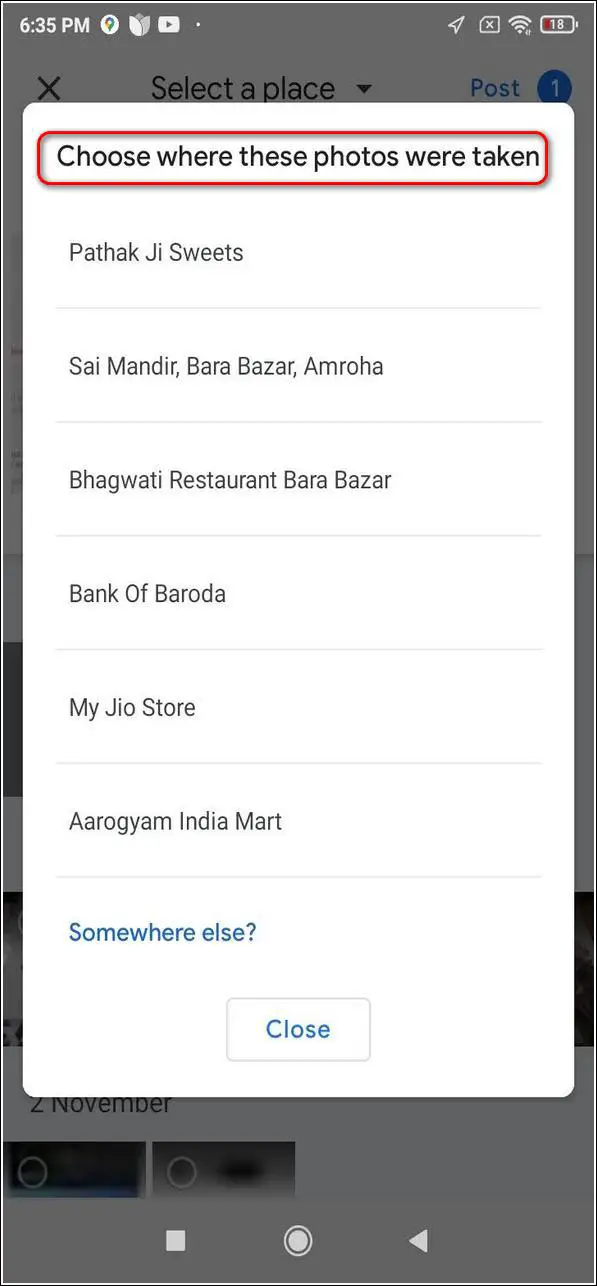On a mobile phone screen, there is a purple-themed pop-up notification taking up the upper part of the display. The notification is rectangular with a black header at the top. The first line of text reads, "Choose where these photos were taken," and is highlighted with a red box outlining it. Directly beneath this, the text "Pataji Sweets" is displayed. Below this display, a thin gray line runs horizontally across the screen multiple times.

Further down, there's a prompt asking "Somewhere else?" alongside a "Close" button. There is an additional box with unidentifiable text.

In the background, the status bar at the top of the phone indicates the time as 6:05 PM. A white circle icon with a gold and pink design is visible, along with a white and gray flower icon. The YouTube app icon can be seen as well. The phone’s battery is shown to be at 18% charge, with the battery icon displayed in red and the percentage in white.